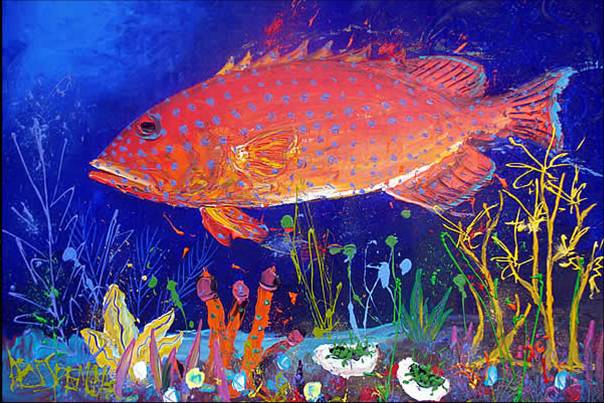This image is a horizontally oriented painting of a large, orange fish with blue spots, swimming from right to left. The fish has dark eyes, fins along the top and bottom, and a tail facing the right edge of the image. Its mouth area and underside have hints of white. The background is a deep, dark blue, representing the ocean, with a variety of colorful ocean plant life on the ocean floor beneath the fish. 

On the bottom right, there are hard-boiled egg-like structures with green pesto, while yellow stick-like plants and dark green foliage are scattered throughout. In the center, there is a patch of orange coral, along with some white and green elements, and a prominent yellow star-shaped plant in the bottom left corner. The artist’s signature is found in bright yellow-green in the bottom left-hand corner, though it is unreadable. The combination of vibrant colors and detailed marine elements makes the image lively and rich in aquatic themes.